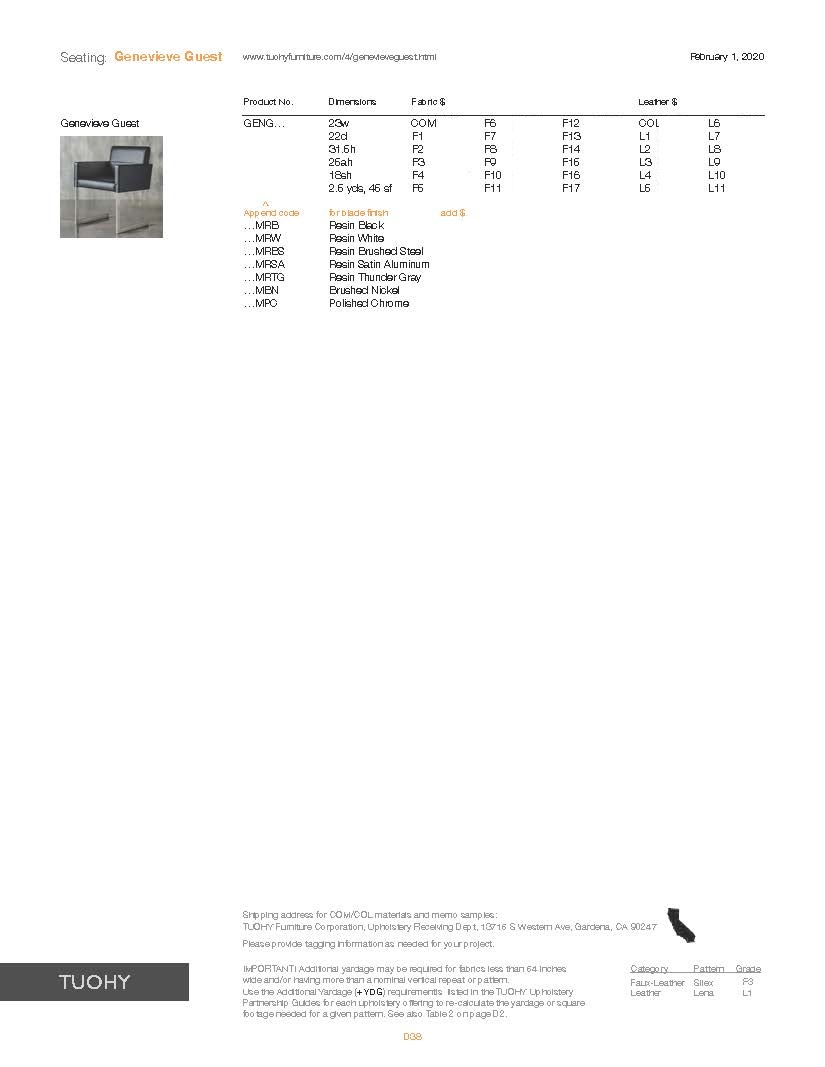Screenshot of a Product Listing for a Tuohy Furniture Chair

This screenshot is from Tuohy Furniture's online catalog, dated February 1st, 2020. The main product featured at the top is labeled "Seating - Genevieve Guest," with the name highlighted in orange. The webpage URL for this product is www.tuohyfurniture.com/4/GenevieveGuest.html.

The listing provides comprehensive details about the chair, including the product number and dimensions (width, depth, height). It appears in a columnar format with six distinct sections that categorize various attributes of the item. 

A photo of the chair is present, showcasing its simple yet elegant design. The chair is made of leather, supported by metallic bars forming L-brackets that run down the front and angle straight back. These metal supports appear to be finished in brushed steel, giving the chair a sleek, modern look.

Additional information includes different finishing options available for the chair, such as resin, aluminum, brushed steel, and color choices like white, black, and gray. A gray rectangle in the bottom lower left corner provides shipping information and details about the item, alongside an outline of the state of California, hinting at shipping origin or destination.

Overall, this screenshot seems to be a catalog entry rather than a purchase page, providing an overview of the product's specifications and customization options offered by Tuohy Furniture.